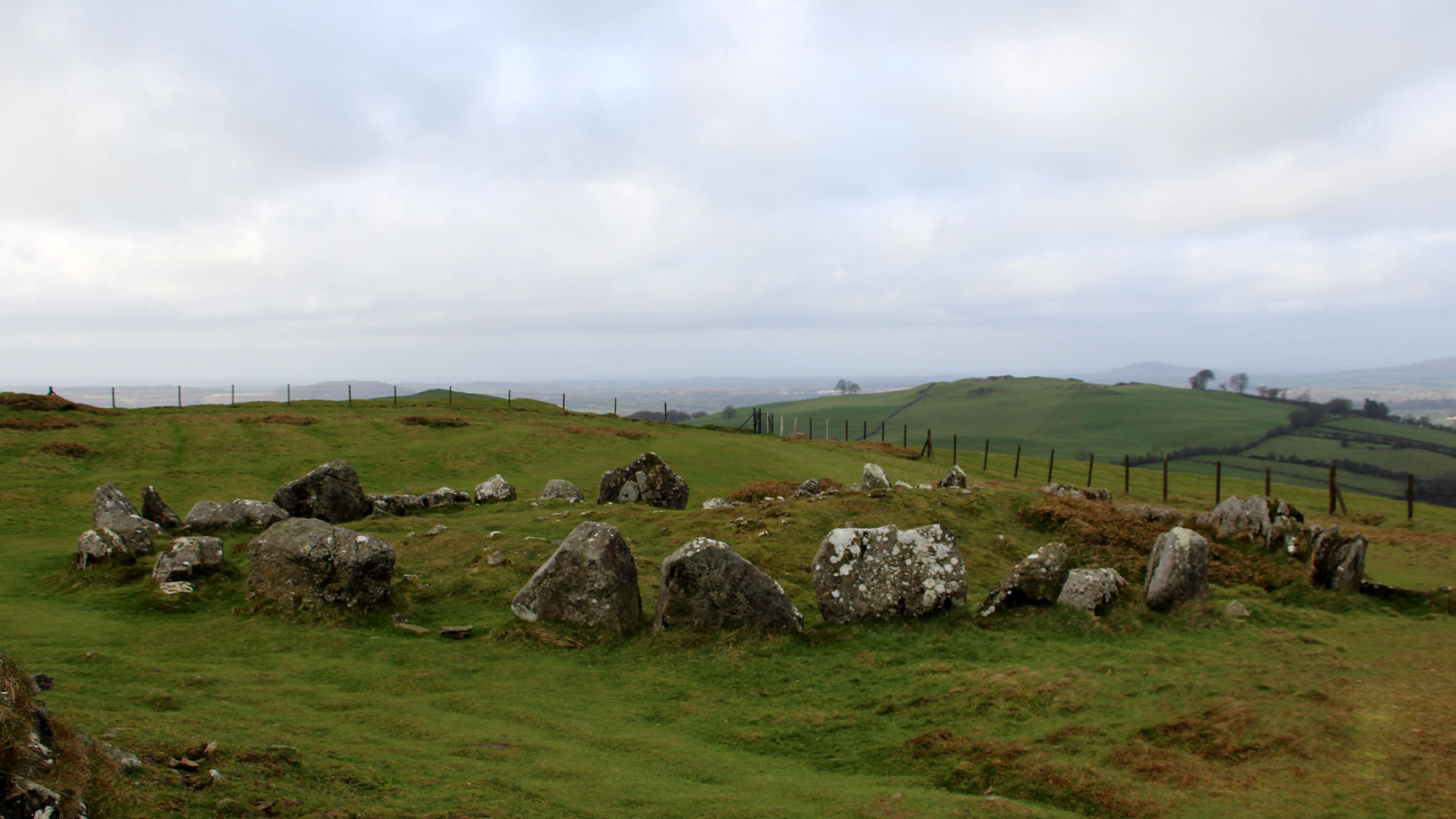The photograph captures a serene countryside scene on a mostly cloudy day. At the forefront, there's a grassy area with some brown patches, particularly on the right, and mostly greenish moss-like grass. Dominating this area is a fairy circle formed by a collection of large, gray stones with white markings that outline a circular raised mound of earth. Beyond this circle, the landscape extends into grassy plains interspersed with wooden fence posts that create a secondary barrier. These fences traverse the image from the left to the right and then curve slightly downward and out of the frame on the right. In the distance to the left, the horizon appears grayish, while more green areas and scattered trees can be seen on the right. The background includes minor hills, some of which are adorned with trees, and far-off, a faint mountain range can be detected. The sky above is predominantly cloudy, adding a somber but peaceful ambiance to the scene.